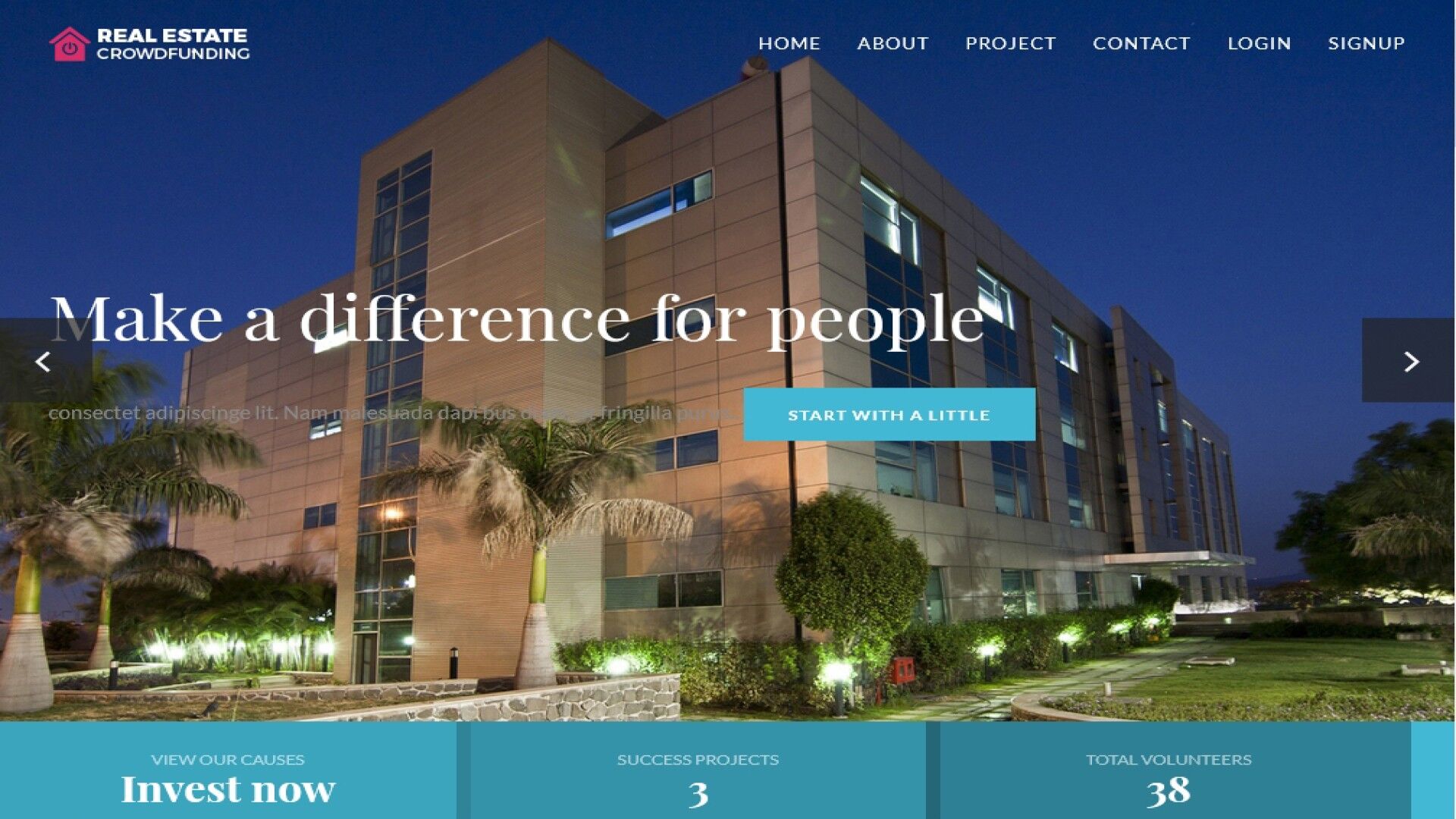This is a detailed screenshot of a webpage from the website "Real Estate Crowdfunding." The logo of the site, which features a house, is prominently displayed and appears in a purplish hue. The top navigation bar includes tabs labeled Home, About, Project, Contact, Login, and Sign Up. Centrally featured on the page is a motivational phrase, "Make a Difference for People," flanked by a left-facing arrow and a sky-blue button that reads "Start with a Little." To the right of this phrase, there's a right-facing arrow.

Below this section are additional tabs: "View Our Causes," "Invest Now," and "Success Projects." Beneath these tabs, informative statistics are displayed: "Total Volunteers" with the number 38, and "Success Projects" listed as 3. The background image is a stunning nighttime shot of a property ensconced by lush landscaping, including palm trees, hedges, and a meticulously maintained lawn. The building elucidated appears to be an office structure, showcased from a corner angle to reveal two entrances and multiple windows. The building's exterior is brown and well-lit with green-glowing spotlights positioned in the surrounding bushes. The overall ambiance presented by the page is inviting and professional, aligning with the theme and purpose of the "Real Estate Crowdfunding" website.